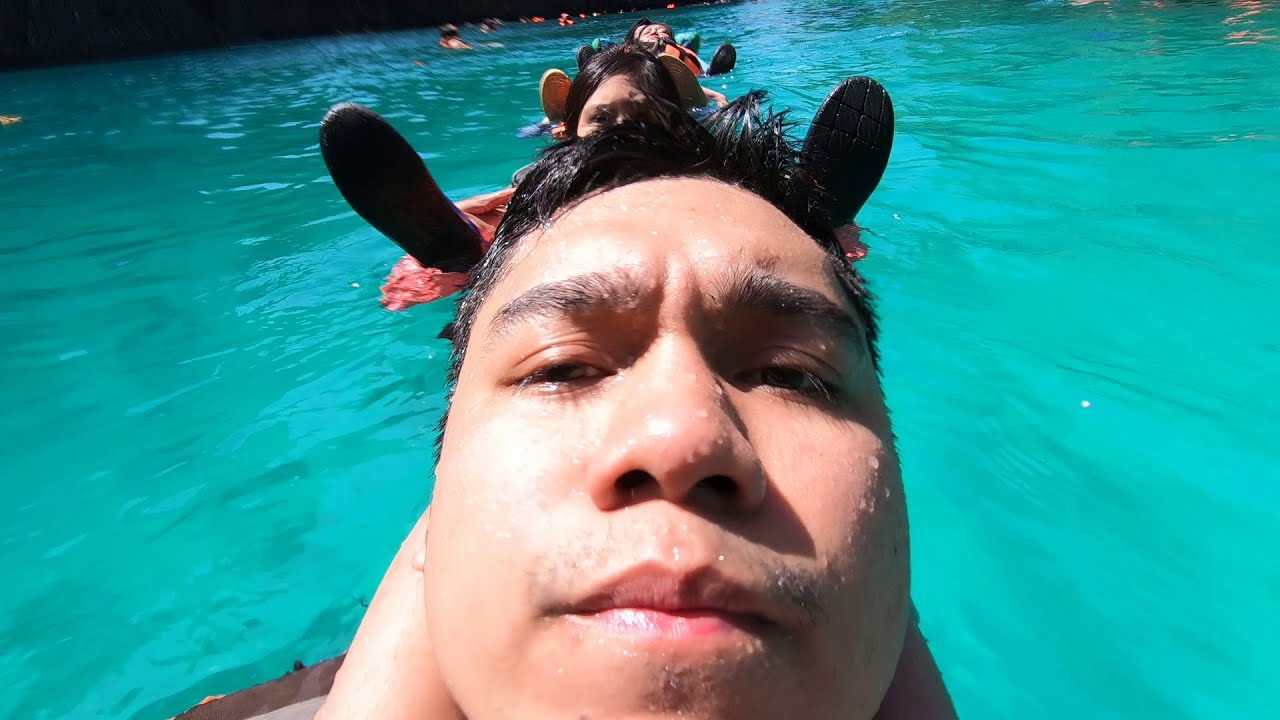The image captures a selfie of a young boy, around 12 or 13 years old, with short black hair and slight mustache stubble, set against the vibrant backdrop of a turquoise or aquamarine-colored lazy river. He has a relatively broad nose, tan to caramel-colored skin, and looks to be of Hispanic or possibly South Asian origin. He fills most of the photograph, with his chin partially cut off. Behind him, a young girl, about 6 or 7 years old, floats on her back with her feet pointing upwards, creating the illusion that her legs are framing the boy’s face like ears. The scene is illuminated by sunlight, casting shadows primarily to the left side of his face, which appears broader due to the camera angle. Around them, several other people float leisurely on the serene water, some in what seems to be orange life preservers. The water is calm but rippled, adding a dynamic texture to the serenity of the scene.